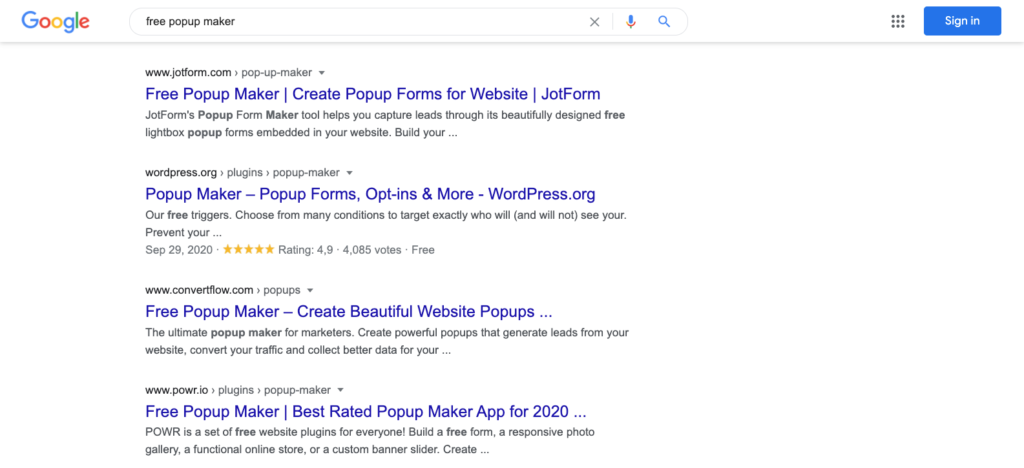The image is a screenshot taken from a computer, depicting a Google search results page. At the top left corner, the colorful Google logo is prominently displayed, featuring the familiar color scheme: blue, red, yellow, blue, green, and red. In the search field, the user has entered "free pop-up maker," with an 'X' icon available to clear the search. Next to it, there is a microphone icon for voice search and a magnifying glass icon for initiating the search. Adjacent to these, the Google apps icon is visible, followed by a blue "Sign In" button.

Below the search bar, the search results are listed:
1. The first result is titled "Free Pop-up Maker - Create Pop-up Forms for Website," linking to jotform.com. A brief description and the website name accompany the title.
2. The second result is "Pop-up Maker - Pop-up Forms, Opt-ins, and More," linked to wordpress.org, with additional information and the website name.
3. The third is "Free Pop-up Maker - Create Beautiful Website Pop-ups," linked to convertflow.com, including a description and the website name.
4. The fourth result is "Free Pop-up Maker - Best Rated Pop-up Maker App for 2020," with information about the app and a link to powr.io (spelled P-O-W-R.io).

The background of the image is predominantly white, with black text for general information and blue highlighted text for clickable search results.